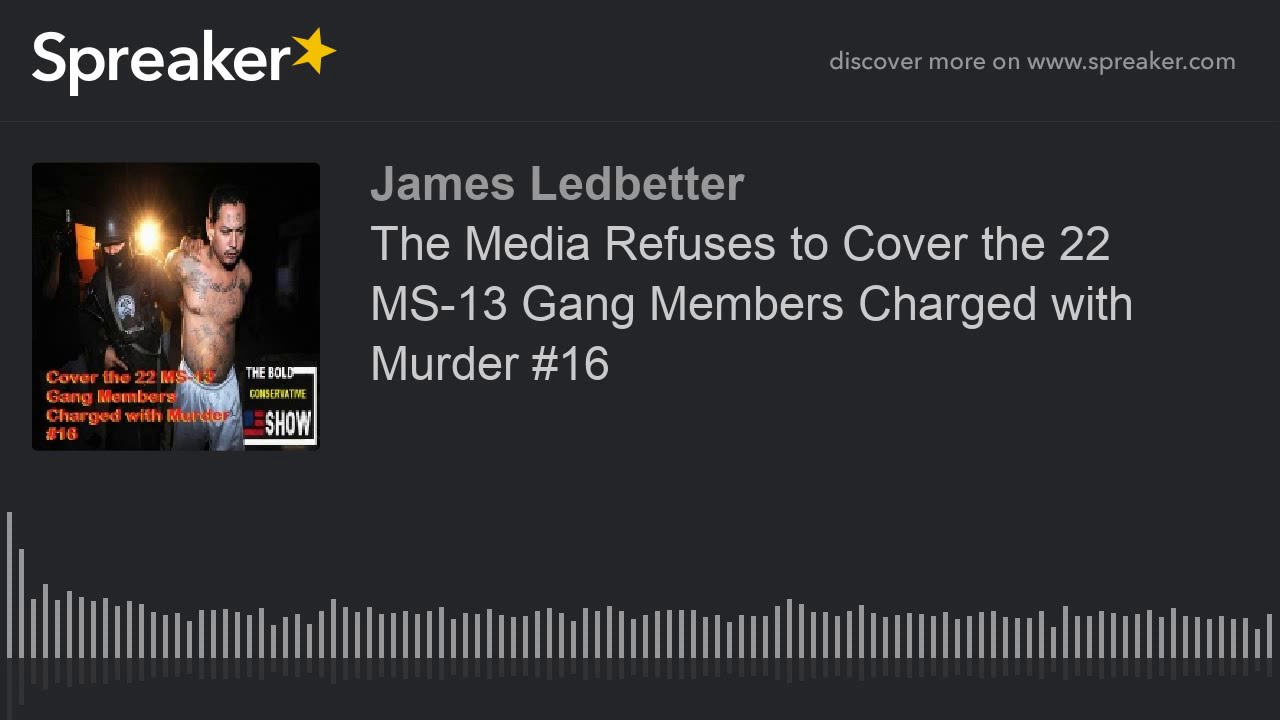The image is an advertisement for a podcast on a dark gray background. In the top left corner, the white text "Spreaker" followed by a yellow star is prominently displayed. On the top right, there is white text that reads "Discover More on www.spreaker.com." The center of the image features white text spanning four lines: "James Ledbetter. The media refuses to cover the 22 MS-13 gang members charged with murder, hashtag 16." To the left, there is a compelling picture of a shirtless man with tattoos being arrested by someone in SWAT gear. Along the bottom of the image, audio bars of various lengths are visible, indicating audio tracking.